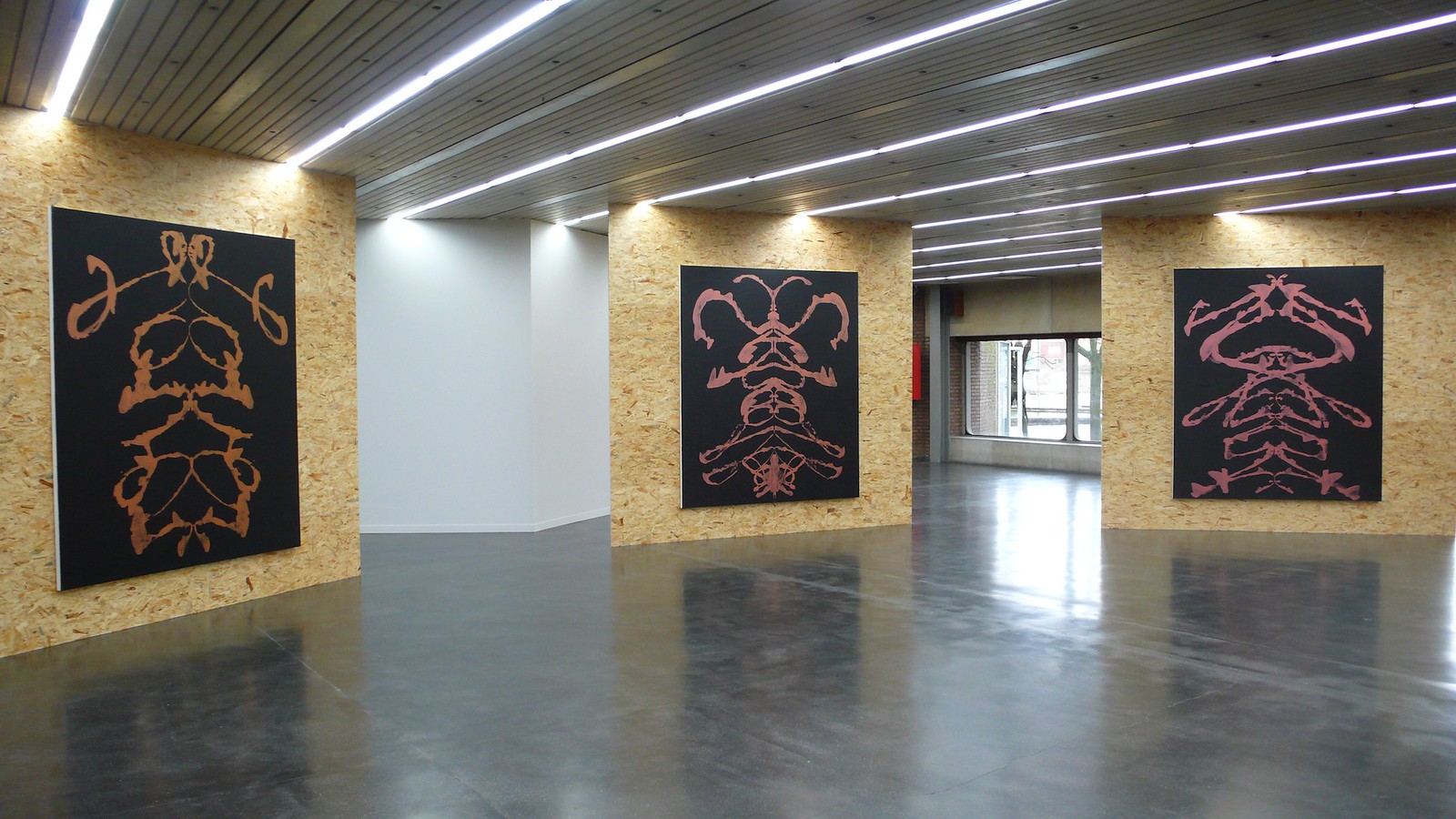This indoor photograph depicts a modern art gallery with a vast, open space. The gallery features a smooth, polished, grayish-black concrete floor and white walls. Suspended above is a ceiling with thin fluorescent lights and metallic planks, enhancing the room’s illumination.

Three large OSB plywood boards stand prominently in the center of the room, each hosting an abstract painting on a black canvas. The painting on the left, characterized by bold orange lines, resembles an abstract insect or a Rorschach test. In the middle, a canvas with a pink outline design portrays an ambiguous form, possibly a bug-like creature with noticeable hooks and eyes. The rightmost artwork, using a different shade of pink, depicts what could be interpreted as an abstract human figure, outlined with suggestive head, torso, arms, and legs features. These paintings, approximately four by six or seven feet in size, stand on plywood boards that extend from the floor to the ceiling, firmly supporting the artworks. In the background, a window offers a glimpse of the outside, contrasting the indoor exhibition space.

Each piece blends abstract expression with thick lines, fostering intrigue and interpretation, reflecting the gallery's embrace of modern art.